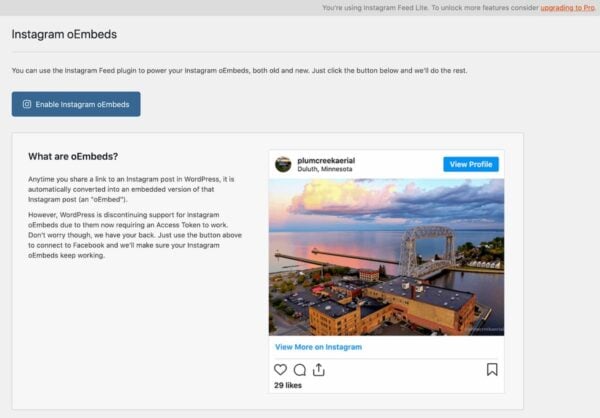The webpage has a minimalistic design with a very light gray background. At the top of the page, a banner reads: "You're using Instagram Feed Light. To unlock more features, consider upgrading to Pro." Below this, there is a section titled "Instagram Embeds," explaining that you can use the Instagram Feed plug-in to manage both old and new Instagram embeds. A blue button labeled "Enable Instagram Embeds" is provided for users to make these adjustments.

The text elaborates that whenever a link to an Instagram post is shared in WordPress, it is automatically converted into an embedded version of that post. However, WordPress is discontinuing support for Instagram oEmbeds, meaning they now require an access token to function. The website reassures users by stating, "Don't worry though, we have your back. Just use the button above to connect to Facebook and we'll make sure your Instagram oEmbeds keep working."

Additionally, there's an embedded Instagram post from Plum Creek Aerial, showcasing an aerial view of a water area, a bridge, and a large building in Duluth, Minnesota. The post has already accumulated 29 likes and includes a prompt to "View more on Instagram."